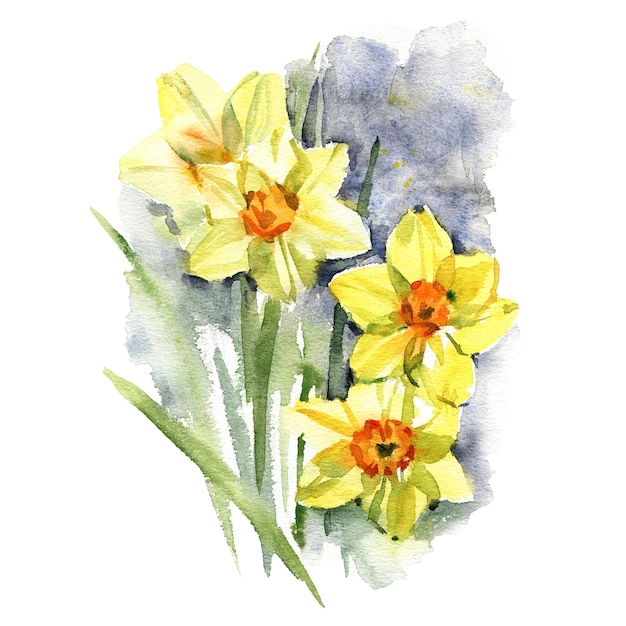This watercolor painting on white textured paper features four bright yellow daffodils with pointed petals, resembling stars. The flowers are arranged with two in the upper left and two in the lower right, each exhibiting a distinctive central disc: an orange center with red around the edge and black dots in the very center, with one flower in the upper left showing a brown center. The painting measures approximately four inches high and three to four inches wide. Detailed leaves and stems in varying shades of green emerge from the lower left corner, depicted as thin, long stalks with pointy blades. The background is a blend of blue and light blue washes, suggestive of a sky, while the upper right and lower right regions are adorned with blotchy shades of gray and purple. The artwork is presented with no visible borders or artist signature, focusing purely on the vibrancy and natural beauty of the daffodils against a serene sky backdrop.